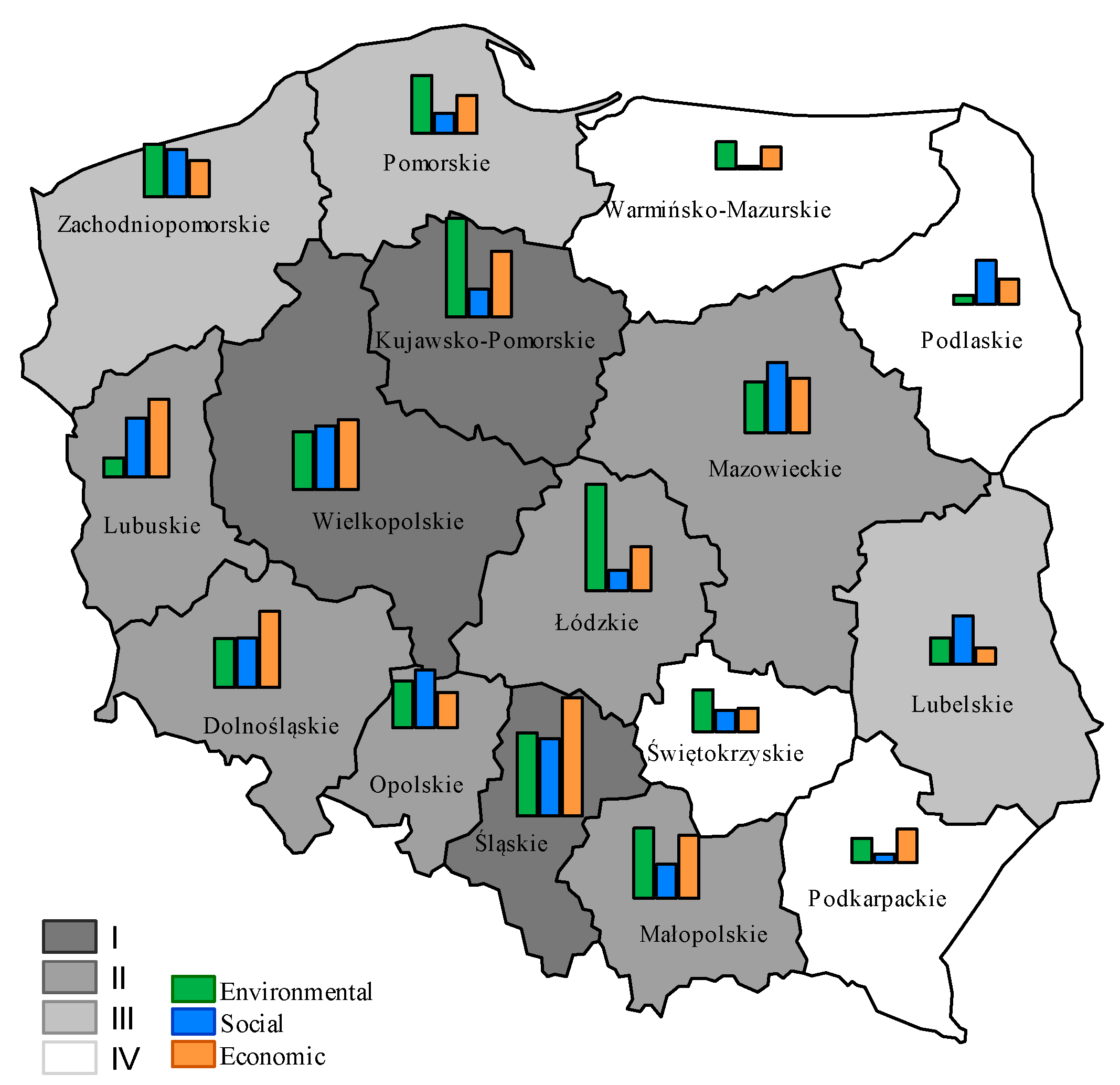This image features a detailed political map, likely representing a country or region once part of the Soviet Union or Poland, given the presence of place names such as Podlaskie, Lodzkie, Slaskie, Lubuskie, and Pomorskie. The map is divided into approximately 20 subregions or states, each demarcated by black borders. 

The regions within the map vary in shading, from white to dark gray, corresponding to a legend in the lower left corner that uses Roman numerals I through IV. However, the specifics of what these numerals represent are not entirely clear. Each subregion also contains a bar chart displaying three bars: green for environmental data, blue for social data, and orange for economic data. The bar charts provide a comparative view of these functionalities across the different states or counties. Additionally, the map contains black text descriptions in a foreign language, likely Polish, indicating the nature and extent of the data within each segment. The overall layout, including the bar graphs and the graded shading, suggests a comprehensive comparison of environmental, social, and economic factors across the various regions.